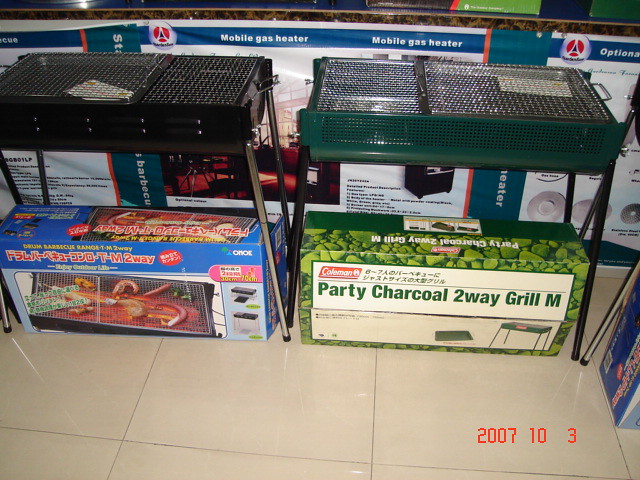In this photograph taken on October 3rd, 2007, the scene is set in a store with a hard tiled floor. The focus is on a display of two charcoal grills positioned side by side. On the right, a green Coleman Party Charcoal Two-Way Grill stands out with its silver grates and text in both English and Asian script on its box, which sits directly beneath it. To the left, another grill, this one black with black grates and four thin silver legs, is perched atop a box featuring Asian characters and an illustration of food being grilled. Promotional materials for a Mobile Gas Heater in blue, red, and white can be seen in the background, enhancing the store’s commercial ambiance. The products are neatly aligned, highlighting their portability and design features.